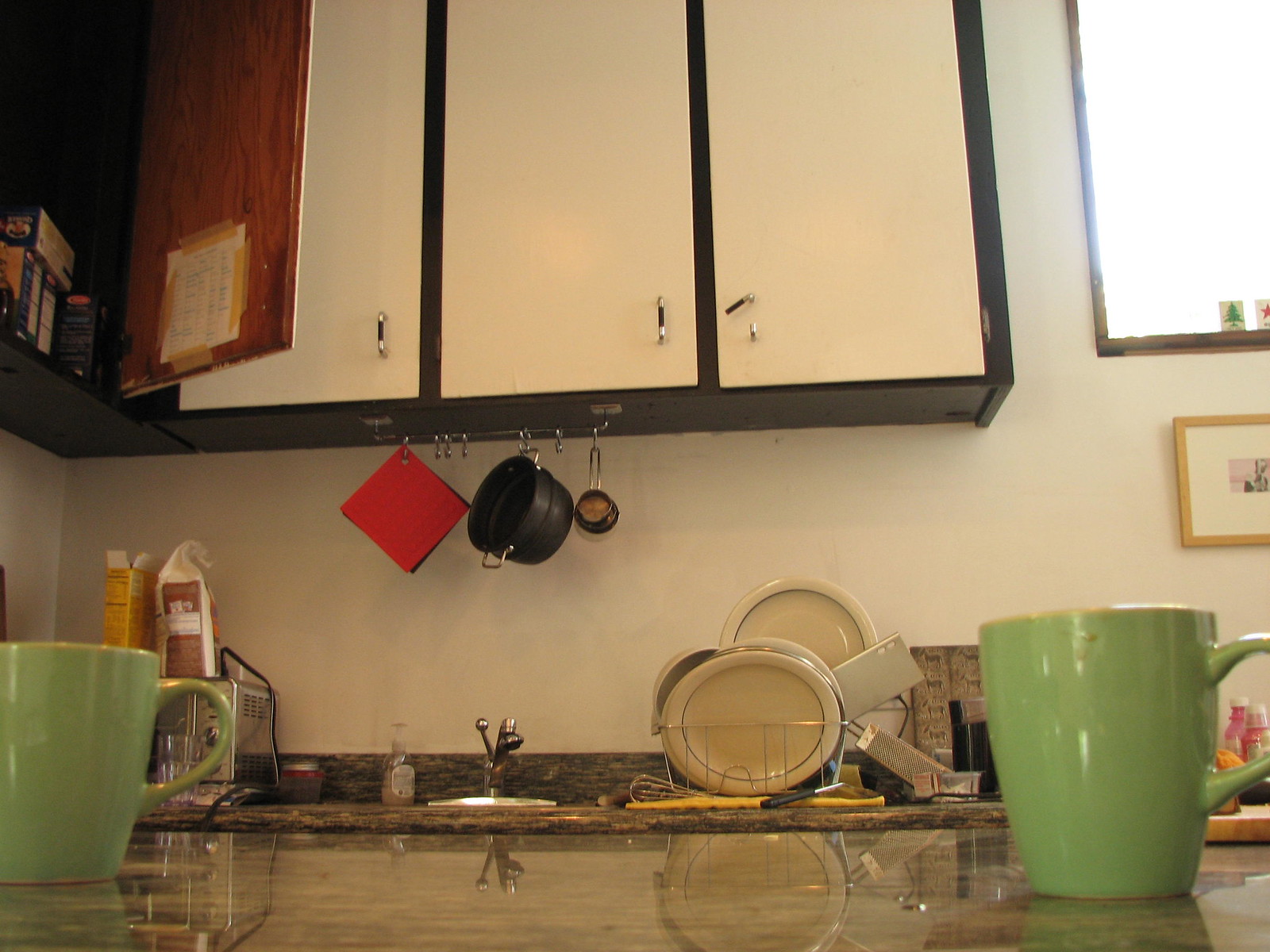This image captures a cozy kitchen scene from the vantage point of a table. The table, which appears to be clean and possibly wooden, features two green coffee cups. The perspective looks up towards the kitchen cabinets, which have a modern two-tone design with white doors and black bodies. The cabinetry spans over the sink and turns left into a corner, where one of the cupboard doors is open, revealing wooden interiors, likely pine, and filled with various boxes that could be macaroni and cheese or noodles.

On the inside of the cupboard door, there is a piece of paper that seems to have frequently called phone numbers. Just to the right of the sink, done dishes are neatly placed in a drying container. To the left, a small appliance that might be a toaster, possibly doubling as a coffee maker, sits on the counter.

Above the sink area, a window allows natural light to filter in, and a small picture is situated just below it on the wall. On the counter beneath the window, there are two bottles with pink contents that resemble Milk of Magnesia, adding a touch of everyday life to the scene. Overall, the kitchen appears well-used and welcoming, with personal touches that suggest it's a hub of activity in the household.